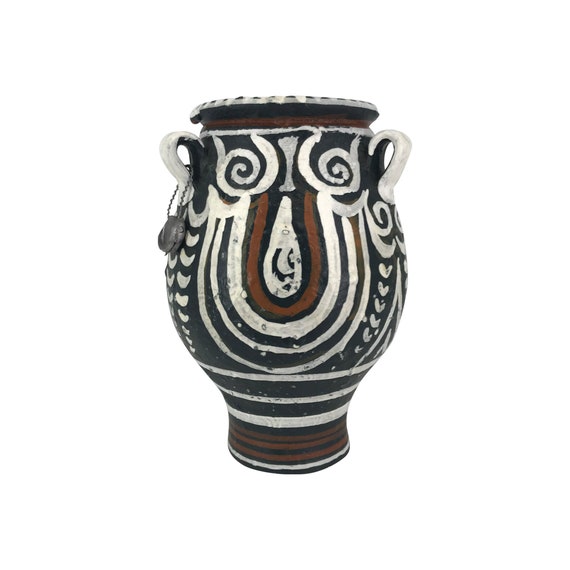The image features an ancient-looking piece of pottery, possibly a substantial decorative urn or vase, characterized by a narrow base that widens significantly at the center before flaring out at the top. The urn is equipped with two white handles on either side, one of which is adorned with a lock and hanging chain. The primary background is black, accentuated by beige and burgundy striped designs along the base and under the rim.

The central painted design depicts an artist's interpretation of a face. The eyes are represented by swirling black patterns, nestled under simple curved white lines denoting cheeks. The nose is highlighted as a large, white, teardrop or raindrop shape. Surrounding the nose are multiple outlines in white, black, and brown, contributing to the intricate detailing. The mouth extends from the teardrop shape into a smiling depiction. Additional features include curved shapes below the handles acting as ears and small, floral-like brush strokes that enhance the detailed artistry of the face. The "neck" area beneath the face is adorned with horizontal spiral patterns, all contributing to the piece's intricate and ancient aesthetic.